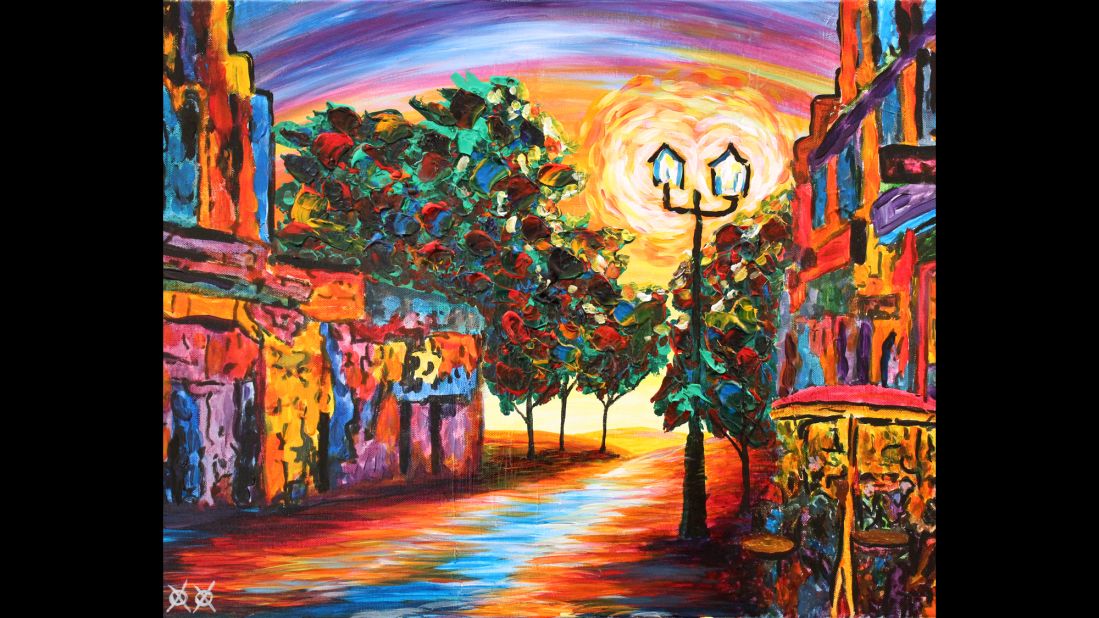This is a horizontal rectangular painting brimming with vibrant, oversaturated colors. The scene depicts a street in a town, framed by thick black borders on either side. The eye is immediately drawn to the center, where a street flanked by buildings stretches toward the horizon. The architecture is alive with reds, blues, yellows, and purples, and each building features tiny balconies. There is an old-fashioned streetlamp with two glowing lamps casting a spectral, jack-o'-lantern-like light, reinforcing the sense of either early morning or late evening. The street itself is divided by a blue central area, bordered by regular paving and red accents on either side. Trees with green and red-blossomed leaves add to the vivid palette and line both sides of the street. In the background, the sky bursts with streaks of deep purples, dark blues, and a rainbow arch of mauve, yellow, and orange, suggesting an enchanted twilight scene. Toward the front right, a cafe scene unfolds with figures in orange, green, and purple, sitting at small tables, adding life and warmth to the surreal, almost hyper-realistic environment.